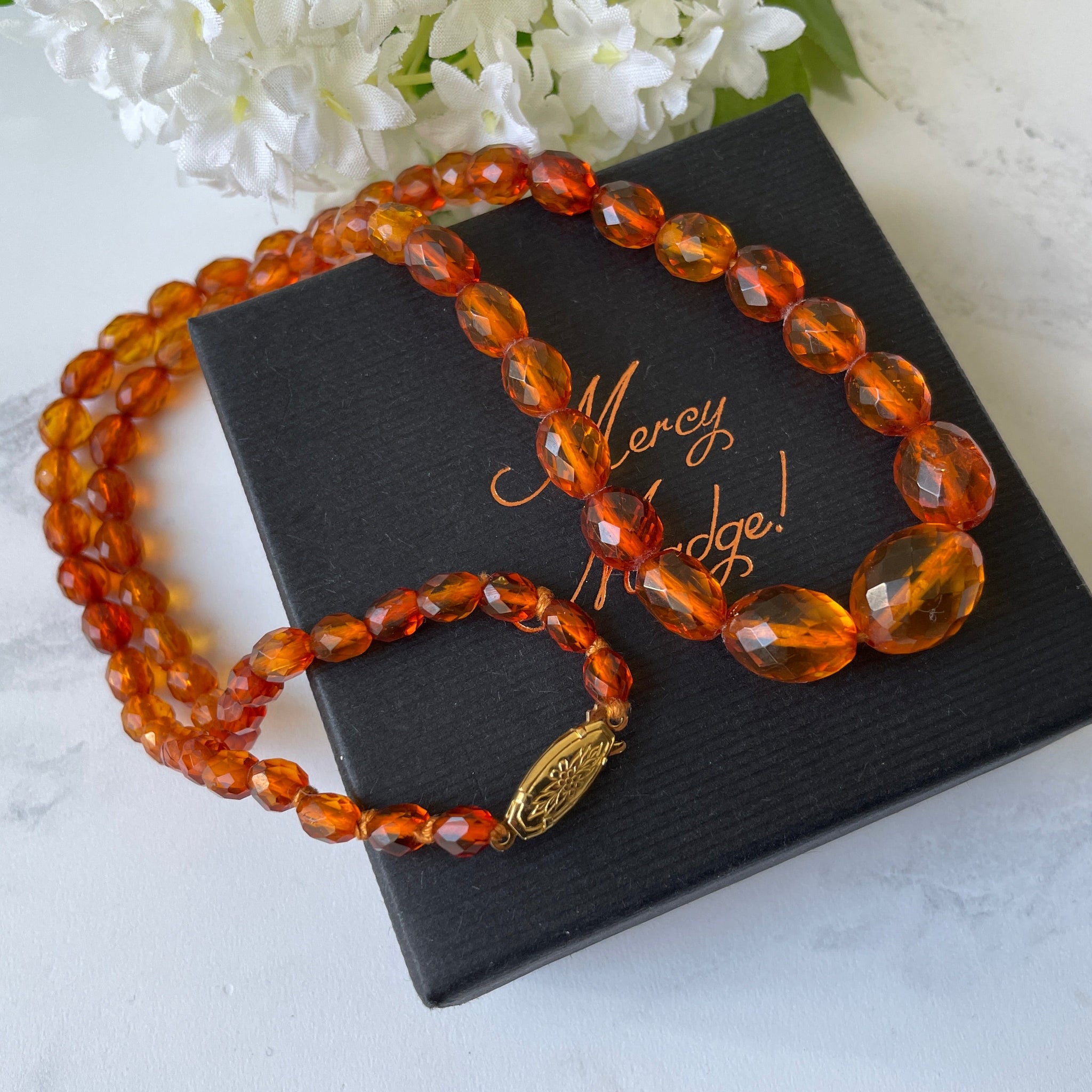This image features a striking orange beaded necklace, appearing to be a thoughtful gift crafted from glass or plastic stones. The oval beads, etched with a faceted texture, are strung on a string and culminate in a gold ornate clasp adorned with a floral pattern. The beads exhibit a gradient size, growing larger towards the center and smaller towards the ends. The necklace is elegantly placed on top of a black jewelry gift box, which partially reveals the name "Mercy Hodge," though some text in the second word is obscured. Enhancing the composition, a small assortment of delicate white flowers rests at the top left of the frame. The entire arrangement is set on a luxurious marble surface, adding a refined touch to the presentation.